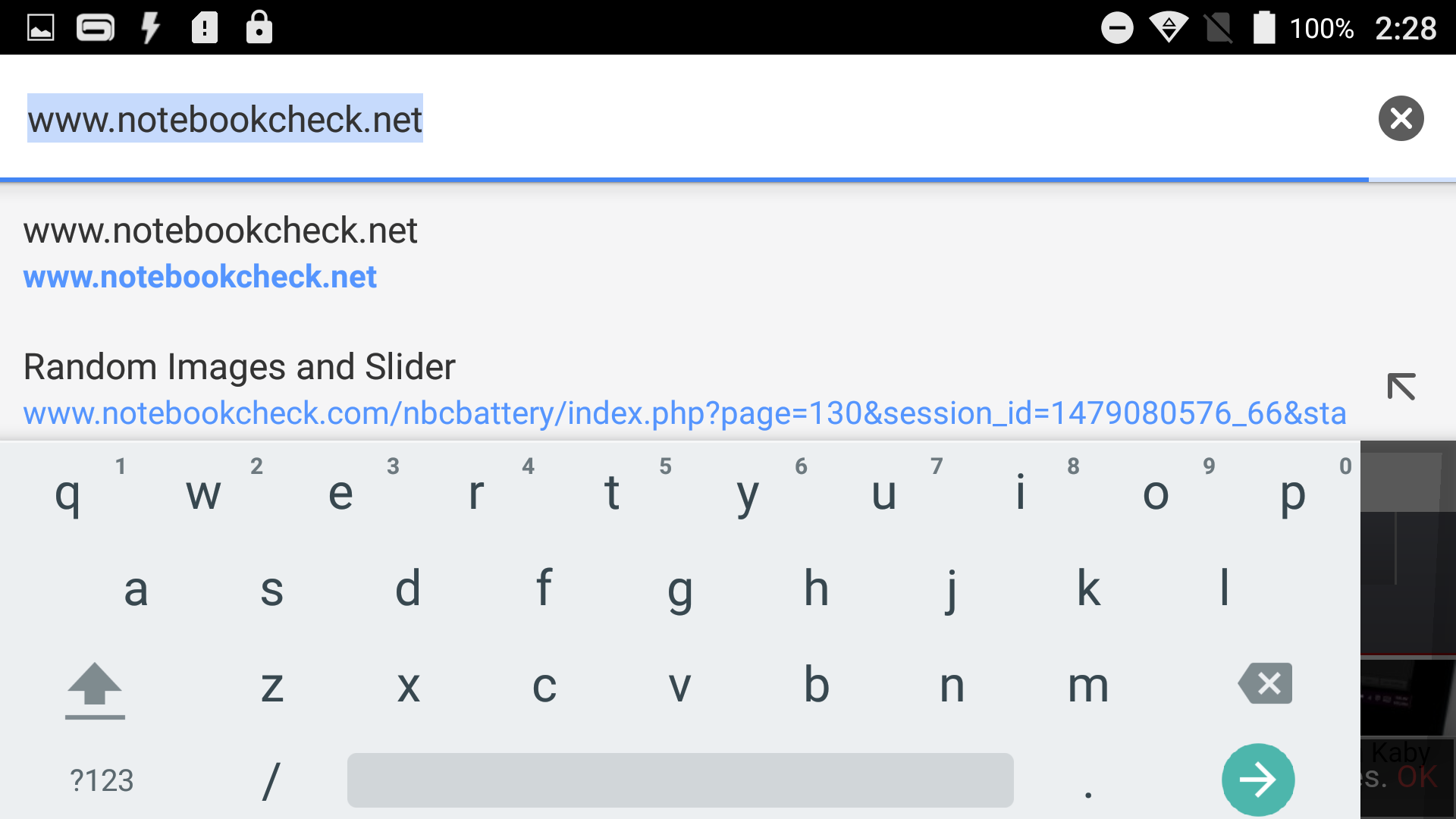A screenshot captured from the website notebookcheck.net displays a web page with various visual elements. At the top of the screen are several icons including a picture icon, a spiral icon, a lightning bolt icon, an exclamation point icon, and a lockbox icon. The battery indicator shows a full 100% charge, and the time is 2:28. 

In the top right corner, there is a circular button with an "X" in it, suggesting an option to close or exit the screen. The URL shown in the address bar is "notebookcheck.net/nbcbattery/index.php?page=130&aspenet_session_ID" and is highlighted in blue.

Below the URL is a light gray keyboard interface with darker gray letters. The keyboard features standard keys including letters, a space bar, a backslash, a period, and a green circle containing a white arrow. An arrow icon points up at the line beneath the keyboard, suggesting an action or direction.